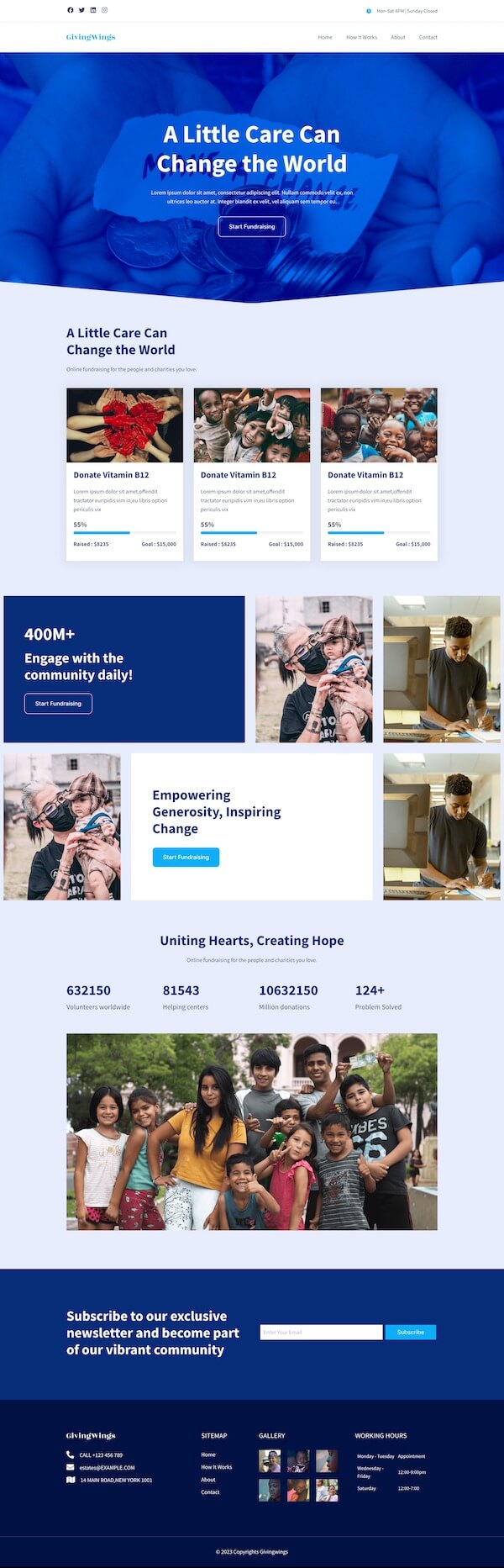The image is a mobile screenshot of a web page featuring a thoughtfully designed layout. The page begins with a translucent dark blue banner at the top. Within this banner, there is a photograph of two outstretched hands, the right hand holding a quarter. Superimposed on this image is a lighter blue blurb with the inspirational white text: "A Little Care Can Change the World."

Below this banner are three smaller photographs, each capturing different moments: the left depicts children's hands, the center shows a group of children, and the right features another group of children, all set against a very light gray background. 

Continuing down the screen, a blue banner proudly declares, "400 million+ engage with the community daily." Following this banner, a white text box reads, "Empowering Generosity, Inspiring Change," accompanied by photographs of a masked woman holding a baby and a man working at a workstation.

Further down, a section proclaims, "Uniting Hearts, Creating Hope," with corresponding numerical statistics. This section also features a long panoramic photo of a group of children, illustrating the impact of the message.

At the bottom of the image, there is a subscribe banner followed by a very dark blue footer containing contact information in white text and six small icons depicting children, tying together the webpage's theme of community and care.